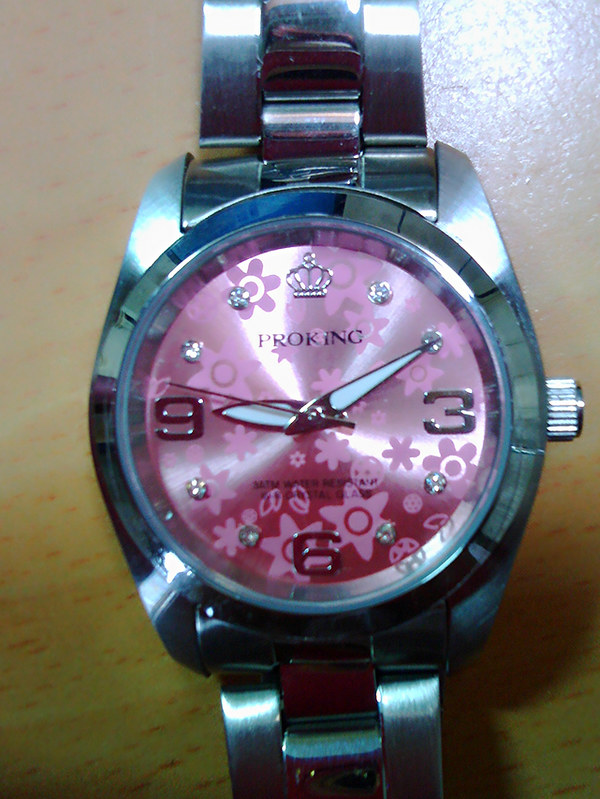This detailed close-up image showcases a luxurious wristwatch with an elegant design. The watch features a robust silver stainless steel case and a distinctive pink dial enclosed under a clear glass cover. The dial itself shimmers with a glossy finish and is adorned with a delicate light pink floral print that adds a touch of femininity. 

Positioned at the 12 o'clock mark is a prominent crown icon, while the hour markers are a blend of silver digits and sparkling diamonds: silver numerals at 3, 6, and 9, and pairs of diamonds for the 1-2, 4-5, 7-8, and 10-11 positions. The brand name, "PRO KING," is displayed in dark pink lettering just below the 12 o'clock crown.

The watch's hands are meticulously crafted; the hour and minute hands are white with silver edging, while the second hand is entirely silver. These elegant hands move over a beige background, enhancing the sophisticated look of this timepiece.